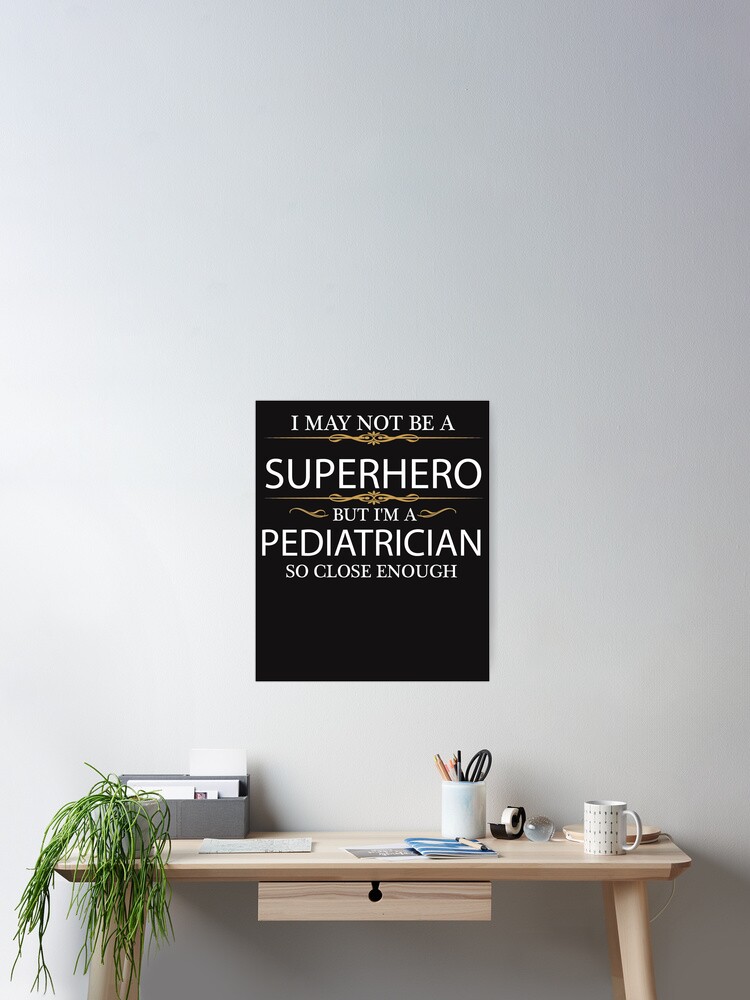This rectangular, vertically-oriented color photograph depicts a minimalist home office workspace with a plain white wall as the background. Centered on the wall is a black poster with white text reading, "I may not be a superhero, but I'm a pediatrician, so close enough," accented with subtle gold filigree patterns. Below the poster is a small, light wood desk with slightly splayed legs and a single drawer with a black handle. 

On the left side of the desk, there's a potted plant with thin, hanging green leaves, accompanied by a gray container possibly holding envelopes or pads. In the center of the desk, a cylindrical holder contains various stationery items such as scissors and pencils, next to a roll of tape. To the right, there is a white coffee mug with dotted accents and an adjustable white desk lamp. The overall setup has a staged, yet neatly organized appearance, making it a compact and functional workspace.